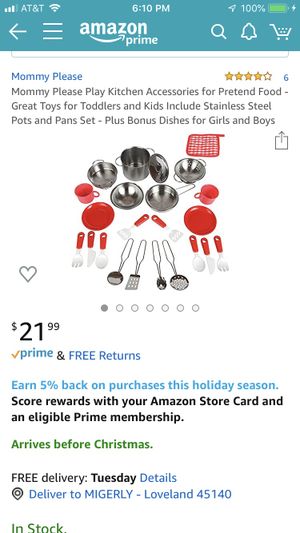This is a detailed caption for the given image:

---

This image is a mobile screenshot from the Amazon Prime app, identifiable by the mobile indicators at the top, including the battery symbol, AT&T signal strength, and Wi-Fi connectivity. The visible product listing is for "Mommy Please" brand, featuring "Mommy Please Play Kitchen Accessories for Pretend Food." The advertisement highlights that the set is ideal for toddlers and kids, including stainless steel pots and pans, along with bonus dishes suitable for both girls and boys. The product image displays multiple pots, pans, cutlery, and other child-friendly kitchen tools. 

In the upper right corner, there is a heart icon for users to favorite the item. The listing shows the price as $21.99, includes the Prime logo indicating eligibility for Prime benefits, and mentions free returns. Below the price, there’s a holiday promotion offering 5% back on purchases made with an Amazon store card for eligible Prime members. The delivery information promises arrival before Christmas, with a specific delivery date of Tuesday mentioned for the address McGear Lee Loveland, 45140. The product is confirmed to be in stock, marked in green font, along with a note about free delivery.

---